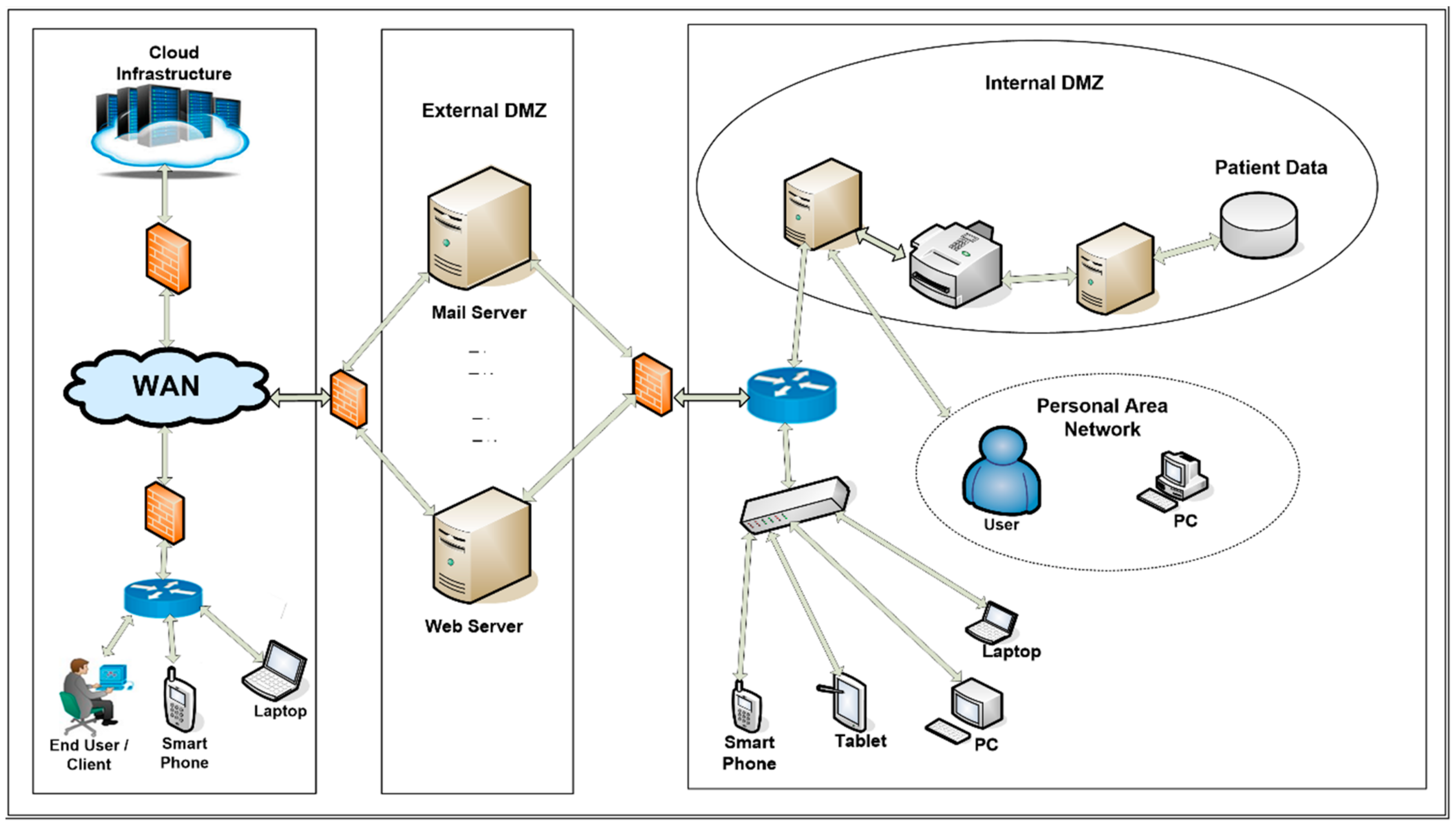This detailed illustration depicts a comprehensive cloud infrastructure setup and communication flow within a workplace. The illustration is divided into three vertically aligned segments on a white background. 

The first segment, labeled "Cloud Infrastructure," features a cloud icon with "WAN" inside it, symbolizing a wide area network. This section shows arrows moving downwards from a cloud that represents the WAN, leading to illustrations of an end-user at a computer desk, a smartphone, and a laptop, signifying different client devices connecting to the cloud infrastructure.

The middle segment is titled "External DMZ" and contains icons representing a mail server and a web server, depicted as computer towers. This section emphasizes the demilitarized zone (DMZ) where external servers reside, serving as an intermediary layer of security.

The third segment on the right, labeled "Internal DMZ," features an oval area containing various computer components such as printers, computer towers, and user devices labeled as PC, smartphone, tablet, and laptop. This segment represents the internal network and includes another oval underneath labeled "Personal Area Network," further detailing the internal setup and user connections.

Overall, the illustration uses arrows to indicate data flow between external and internal networks, highlighting the structured communication pathways from individual devices through the WAN to the cloud infrastructure.